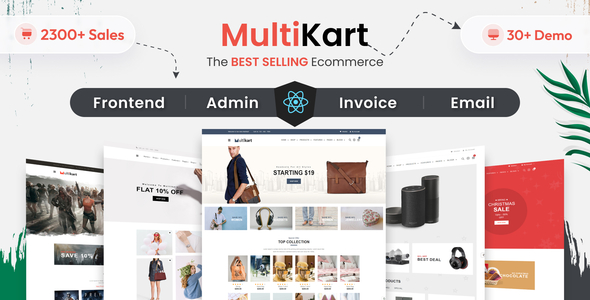This advertisement showcases Multi-KART, a best-selling e-commerce platform. "Multi" is highlighted in bold red letters, while "KART" is displayed in black bold letters. The background is predominantly gray. An arrow extends from the "T" in "KART" to a button labeled "30+ demos." Below it, a tagline announces "The best-selling e-commerce."

On the left-hand side of the ad, there’s an illustration of a grocery cart with the text "2,300+ sales" in orange. This text connects with labels that read "front-end," "administration," "invoice," and "email."

The center of the ad features a nuclear symbol with multiple rings encircling a central dot, symbolizing the core features and comprehensive nature of the platform. Surrounding this central graphic are various icons and images representing different product categories available within the e-commerce platform. These include items such as a purse, headphones, backpacks, clothing, electronics, slippers, and movies.

The clear and dynamic visuals emphasize the multifaceted functionality and extensive sales reach of Multi-KART, making it a compelling choice for e-commerce businesses.